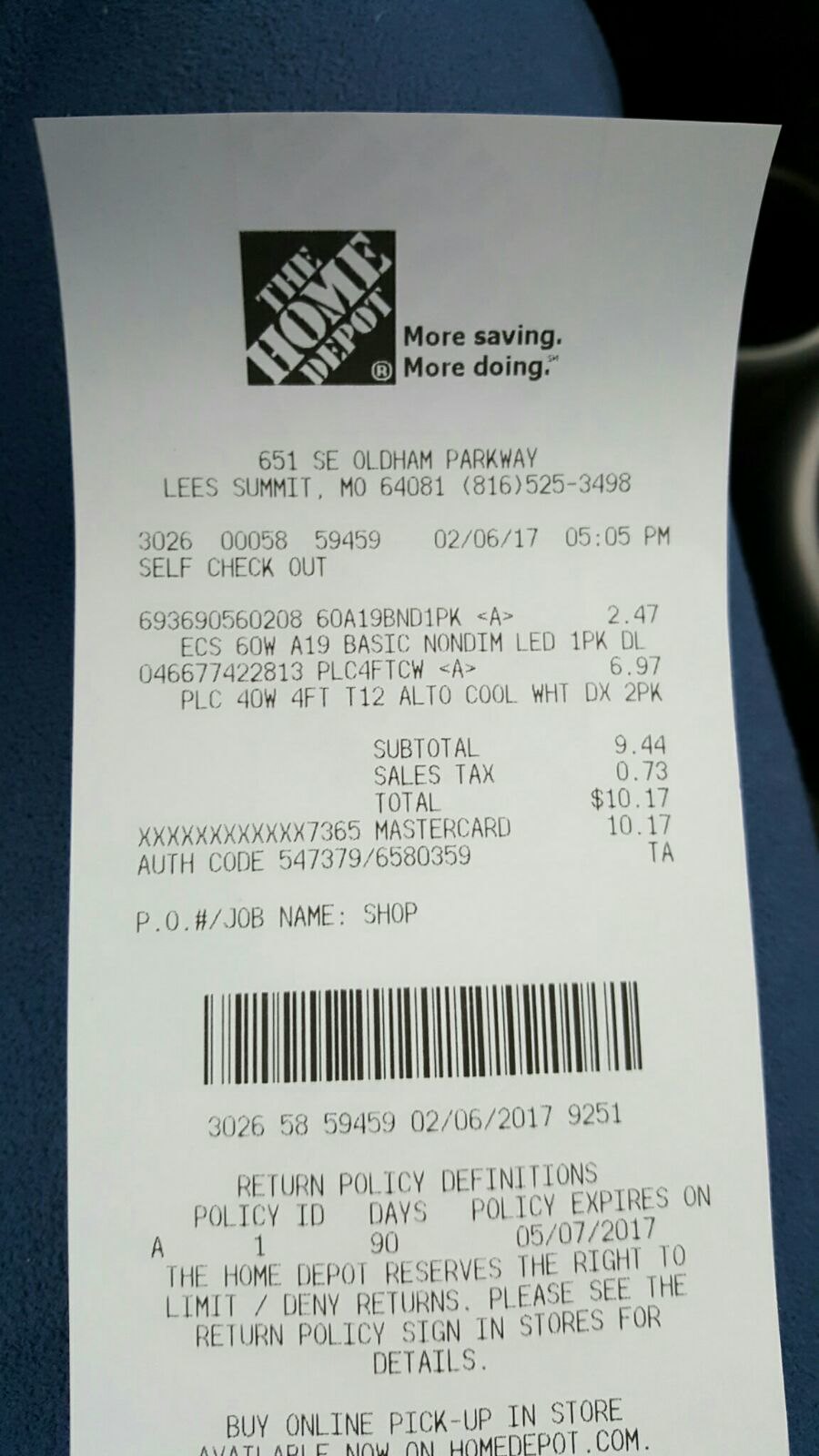This image shows a detailed Home Depot receipt, held up against a medium to dark blue background, likely a piece of furniture. The receipt is from the Home Depot store located at 651 SE Oldham Parkway, Lee's Summit, Missouri 64081, with the contact number 816-525-3498. The top left corner features the Home Depot logo, a black square with "The Home Depot" written diagonally in white, accompanied by the tagline “More saving. More doing.” beneath it. 

The receipt is dated February 6th, 2017, with a timestamp of 5:05 PM, indicating it was processed via a self-checkout register. The purchased items are listed with details: a basic non-dimmable LED pack and a 4-foot T12 Alto Cool White two-pack, priced at $2.47 and $6.97 respectively, leading to a subtotal of $9.44. Including $0.73 in sales tax, the total amount came to $10.17, paid using a MasterCard ending in 7365. The document also includes an authorization code and a barcode for scanning, reiterating the receipt information such as the receipt number, register number, and date.

Beneath the purchase details, the receipt outlines Home Depot's return policy, specifying that returns must be made within 90 days, which would be by May 7th, 2017. The receipt is white with black text, clearly displaying all printed information.